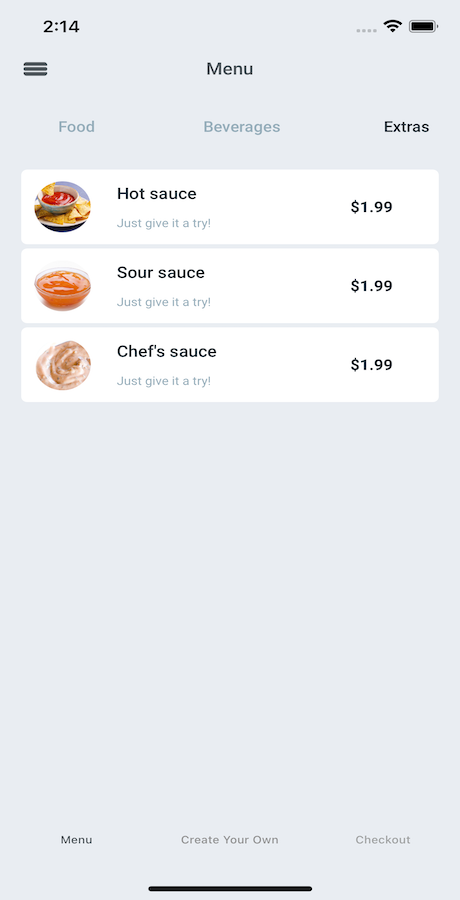The image features a light grey background. At the very top, the number "214" is displayed in black print. To the right, there is an indicator showing the cell signal or WiFi signal, followed by the battery icon and four small, darker grey dots. 

Below, three horizontal lines are stacked on top of one another, each line separated by white space. At the center of this section, the word "Menu" is prominently displayed with a capital "M." 

Continuing downward, the items "Food," "Beverages," and "Extras" are listed horizontally, each word beginning with a capital letter. "Food" and "Beverages" are in light grey, while "Extras" is in black.

Three white panels are shown next:
1. The first panel reads "Hot Sauce" in black print, followed by the phrase "Just Give It a Try" in grey print. An accompanying image of the hot sauce is displayed, along with the price "$1.99."
2. The second panel displays "Sour Sauce" with a picture of the sauce in a bowl and the phrase "Just Give It a Try" in grey print, priced at "$1.99."
3. The third panel features "Chef's Sauce" with a capital "C," an image of the sauce, the phrase "Just Give It a Try" in grey print, and the price "$1.99."

At the bottom of the image, there are options listed: "Menu," "Create Your Own," and "Check it Out" with a solid black line running through the center.